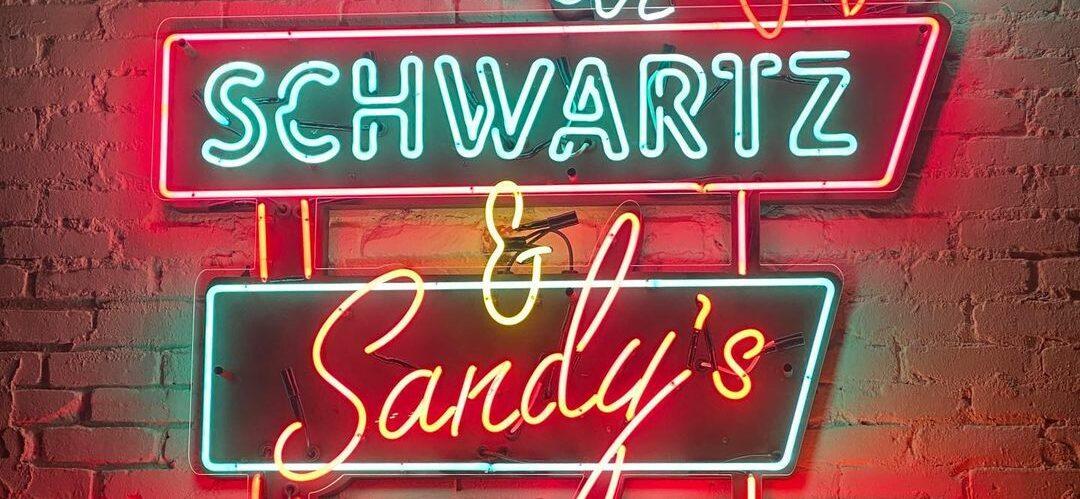The photograph features a detailed close-up of two neon signs mounted against an old brick wall with numerous mortar patches. The image appears to be taken indoors. The primary focus is on the neon signs at the center of the composition. 

The top sign is a red neon-outlined rectangular shape, with a unique extension on the top right, creating a stylized look. Within this red border, the word "Schwartz" is prominently displayed in blue neon light, spelled out as S-C-H-W-A-R-T-Z. 

Suspended below this is a bright yellow neon ampersand (&) sign that connects to the smaller, lower sign. The bottom sign mirrors the design of the top, with a yellow cursive text spelling out "Sandys," extending further on the top right than on the bottom right. The yellow cursive text is bordered by blue neon light. 

The overall effect of the neon lights casts a colorful glow against the aged brick wall, creating a vivid contrast between the modern signage and the rustic background.